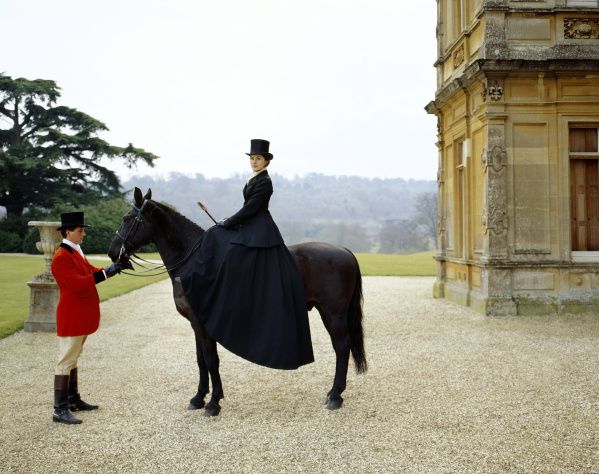The image depicts a striking scene of a woman riding a dark brown horse, almost black in areas, positioned near the center to the left of the frame. The woman exudes elegance, dressed in a long, flowing black dress that nearly touches the ground, complemented by a black jacket, gloves, and a black top hat. She gazes directly at the camera. In front of the horse, a man steadies the reins. He is adorned in a red jacket, black top hat, and khaki pants, along with black leather boots. The background features a mix of natural and architectural elements: to the right, a yellowish concrete building with columns reminiscent of a castle, and to the left, a grassy area with trees. A birdbath or statue is visible behind the man, and the ground appears to be a paved, light gray or gravel surface. The man focuses his attention on the horse.